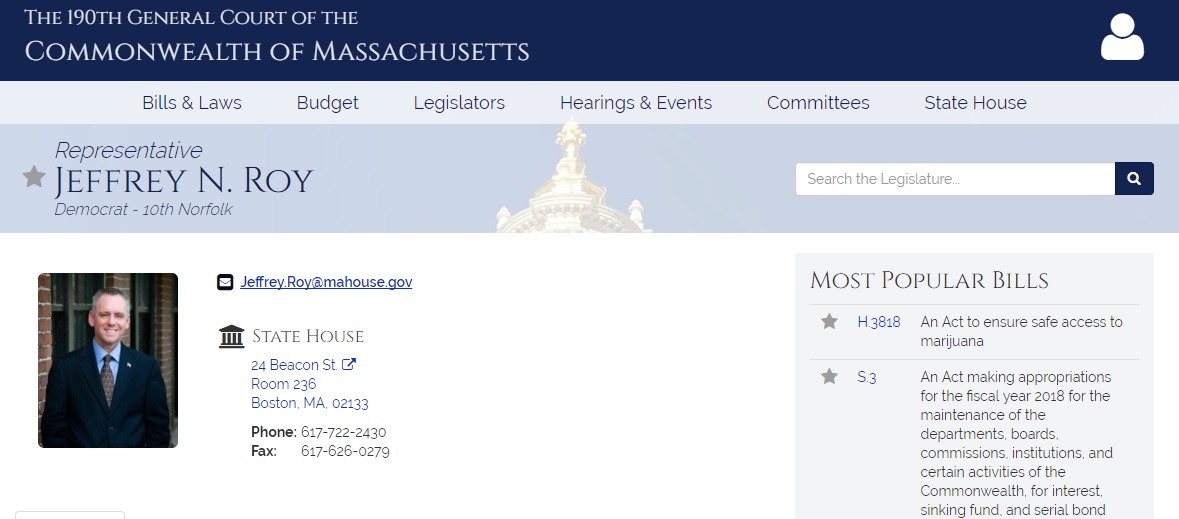This is a detailed screenshot from the official website of the 190th General Court of the Commonwealth of Massachusetts. The primary focus of the image is Representative Jeffrey N. Roy, a Democrat serving the 10th Norfolk district. His photograph is prominently displayed on the left side of the screenshot. Adjacent to his picture, you can find key contact information, including his email address, the address of his State House office, his business phone number, and his business fax number.

At the very top of the webpage, there is a navigational menu with various options such as 'Bills and Laws,' 'Budget,' 'Legislators,' 'Hearings and Events,' 'Committees,' and 'State House.' Below the 'Committees' and 'State House' options, there is a search bar labeled 'Search the Legislator,' accompanied by a magnifying glass icon for executing the search. 

Further down, immediately below the search bar, the site highlights the two most popular bills currently under consideration. The first bill is H.3818, titled "An Act to Ensure Safe Access to Marijuana," and the second is S.3, which pertains to budgetary measures for the state. The structured layout and the detailed information provided aim to offer comprehensive insights and facilitate easy navigation for users interested in legislative activities and representatives.